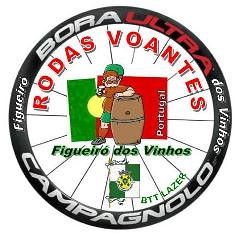The image depicts a circular logo with a white interior and a thin black outline. Central to the design is an illustration featuring a figure that resembles a man with a mustache, possibly of Caucasian appearance, holding a beer while leaning on a brown barrel. The man appears in front of a background that includes a red and green flag, likely indicative of Portugal.

The top of the logo features red text on a white background reading "Rodas Vontes," while below the central image, green text states "Figurito dos Vinhos." A small green and white flag is also present beneath this text. Encircling the entire design, a thin black border contains the phrases "Bora Ultra," with "Bora" in white and "Ultra" in red. The logo likely serves as an advertisement or branding for Portuguese products or events, possibly related to wine or beer.